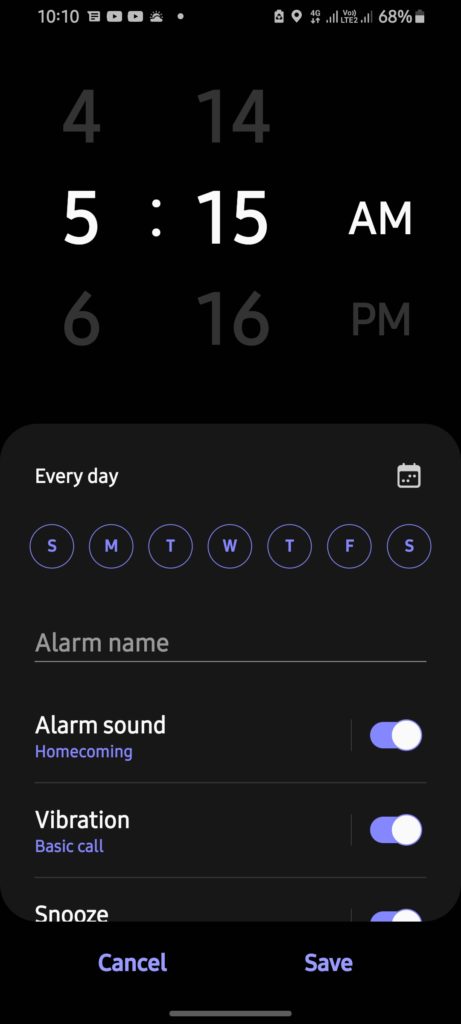This is a detailed screenshot of a smartphone interface. The top half of the image features a primarily black background, transitioning to a dark gray background about an inch from the bottom. The phone status bar spans the top section in black with various icons and information. Starting from the top-left corner in white text, the time is displayed alongside a message icon followed by two icons resembling the Yahoo or YouTube play buttons. A partially cloud-covered sky or sun icon, a small white dot, and the battery charging icon are visible with "68%" next to it. Signal strength indicators show three or four bars for the internet, labeled "LTE", followed by a similar signal with the "4G" label, and arrows pointing up and down to signify data transfer. A location icon is also present.

Beneath this status bar on the gray background, "4" is displayed on the left with "14" on the right. Below this, large white numbers show "5:15 AM" with smaller gray numbers "6:16 PM" adjacent to it.

The subsequent dark gray area lists "Bolded every day" in white at the top-left corner, accompanied by a calendar icon on the right. Below this, there are black circles with purple borders containing the letters: "S", "M", "T", "W", "T", "F", "S" representing the days of the week.

Following a small gap, the gray text "Alarm name" is bolded with a line underneath it. Below it, "Alarm sound" in bold white is followed by the description "Homecoming" in purple, indicating the alarm is toggled on with half the toggle button purple and half white. Next, the word "Vibration" in white is visible, labeled as "Basic Call" and toggled on. Moving further down, "Snooze" in white text partially appears along with an incomplete toggle switch.

In the black portion at the bottom, "Cancel" in purple text is positioned on the left, while "Save" in purple is on the right. In the middle of this section lies a small gray bar, dividing left and right sections.